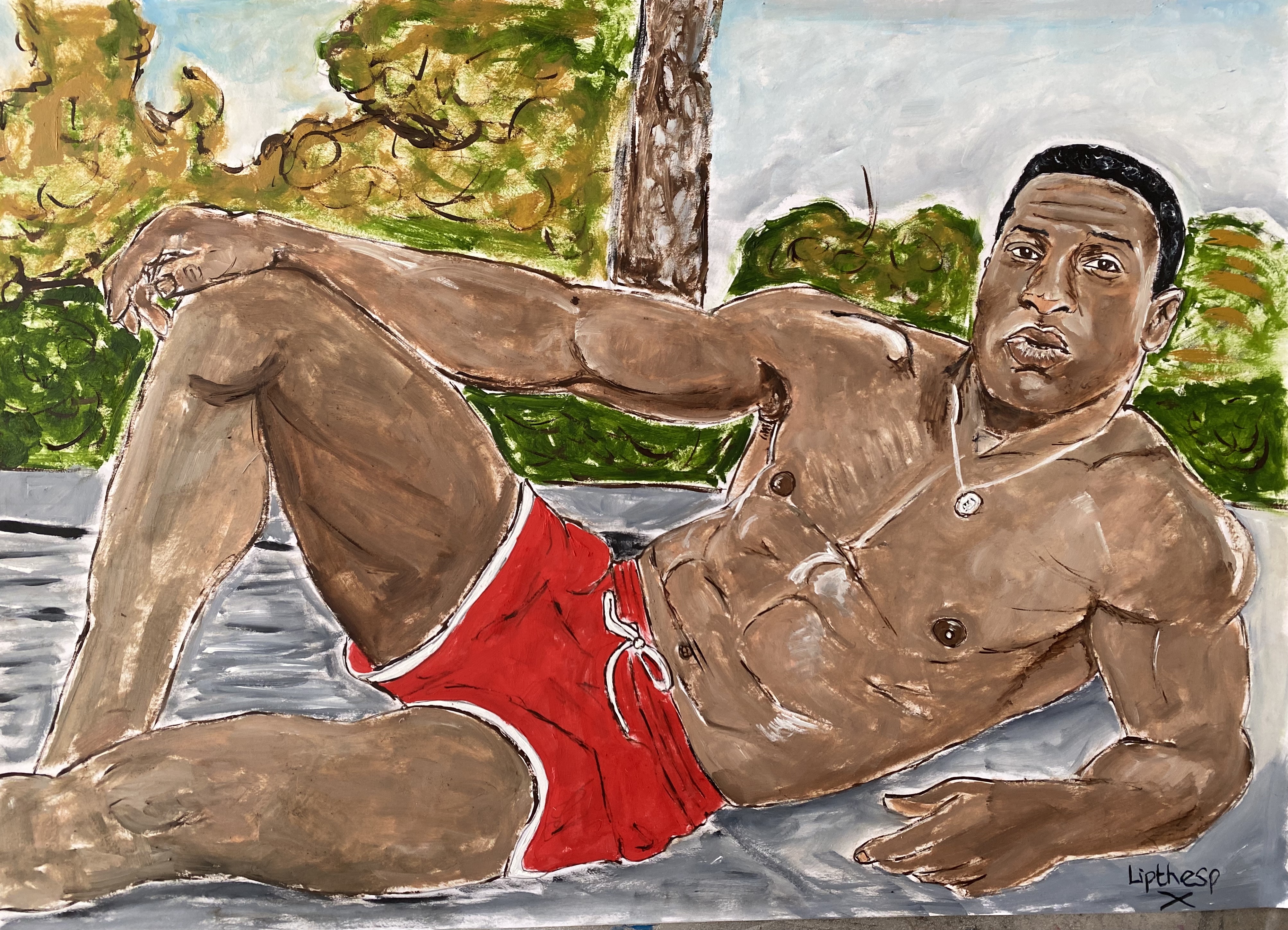The image is a detailed photograph of a painting that depicts a black man lounging comfortably, shirtless, and resting on his left elbow and hip. His body faces forward and his right knee is bent with his right hand draped over it. He's clad in red shorts featuring a white tie on the waistband and white stripes along the legs. Around his neck, he wears a white necklace adorned with a white pendant. The setting behind him includes a lush green forested area with a solitary tree, some shrubs, and a gradient of various green hues, browns, and hints of yellow for shading. The lounging figure reclines on a gray surface, which could be a mat or a float. The painting is signed at the bottom right corner with the name "LIPTHESP" in black, accompanied by a black "X" beneath it. The color palette of the painting comprises browns, whites, reds, greens, grays, and touches of yellow.